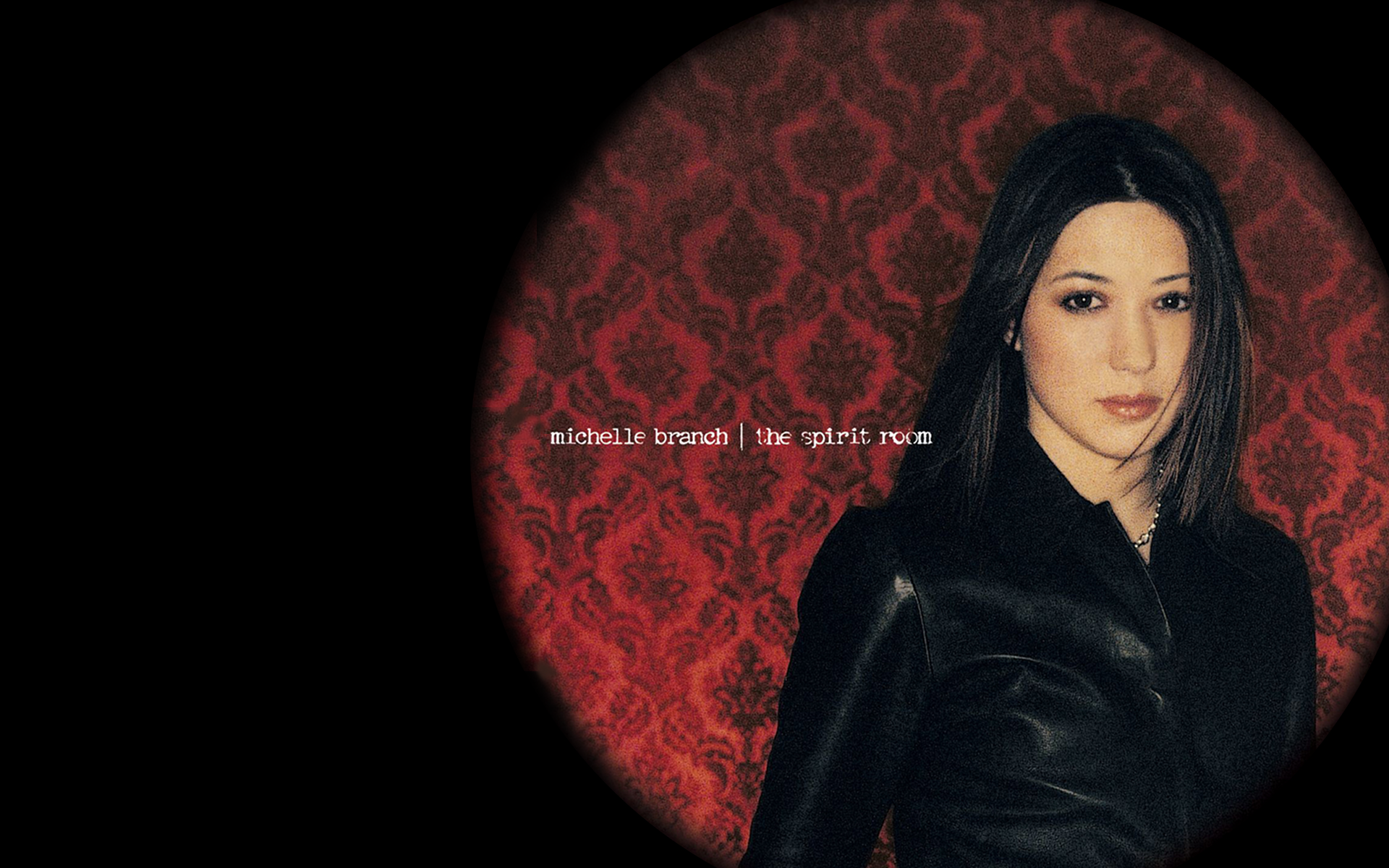The image features a black background with a prominent, circular, red floral-patterned backdrop on the right side. At the center of the image stands a woman identified as Michelle Branch. She is framed from her mid-waist up, looking straight into the camera with an expressionless face. Michelle is wearing a black, zip-up leather jacket with a collar and a silver necklace visible where the zipper ends. Her long, straight black hair reaches her shoulders with a slightly jagged part in the front. She has dark eyebrows, dark eyes, and is wearing red lipstick. To the left of her, in small white text positioned around the bottom-right side of her hair, it reads "Michelle Branch | the spirit room," suggesting this could be an album cover for her work, "The Spirit Room."